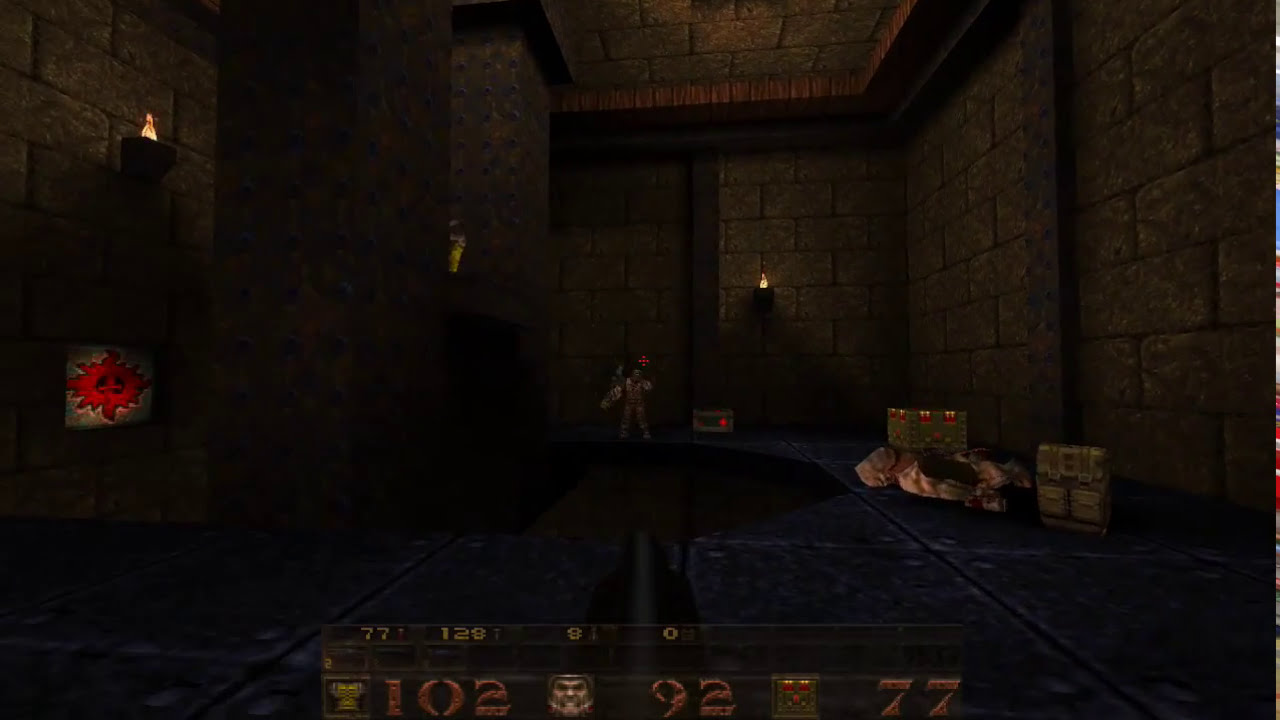This image is a dark, underexposed screenshot from an early 2000s or late 1990s first-person shooter video game characterized by its cartoonish graphics. The scene is set in a dimly lit dungeon or temple with massive stone walls and ceiling. The player's perspective shows them holding a weapon, aiming through a small red crosshair at a figure in the background that resembles a monster or mummy. The room is adorned with various game elements including large bricks, fire-lit lanterns, sconces illuminating parts of the scene, and a miscellaneous pile of game items such as cloth bags, a backpack, and a box. The Heads-Up Display (HUD) at the bottom of the screen shows crucial game stats: 102 armor, 92 health, and 77 ammunition. It also features a character's face and additional game information, reminiscent of the HUD style in classic games like "Doom."